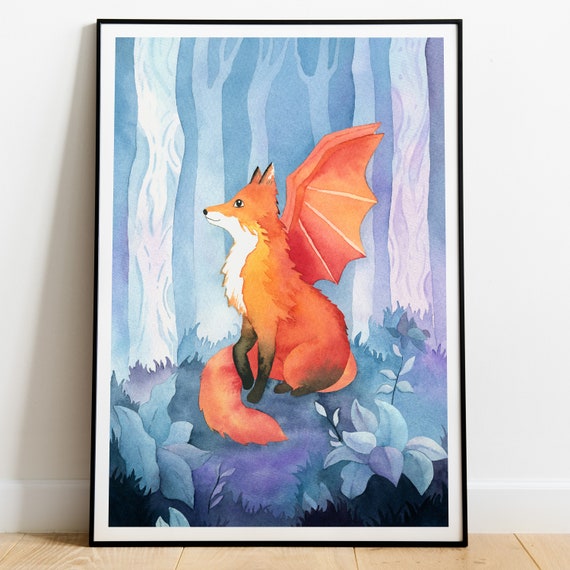The image showcases a captivating watercolor illustration centered on an imaginative portrayal of a fox. The fox, predominantly orange with a white chest extending to its chin and nose, has black fur on its paws. It sits gracefully on its hind legs with a bushy, curled tail wrapped around its legs. Displaying a magical touch, the fox is adorned with orange dragon wings. The illustration breathes life with a vibrant backdrop of bluish-green tinted grass and an array of flowers and plants. Surrounding the fox are stark white trees, indicating it is nestled within the woods. This dreamlike scene is bordered by a white edge and a black frame, leaning against a beige brown wooden surface of an indoor setting, against a white wall. The overall rectangular composition captures a whimsical and detailed vision, perfect as a creative children's illustration.